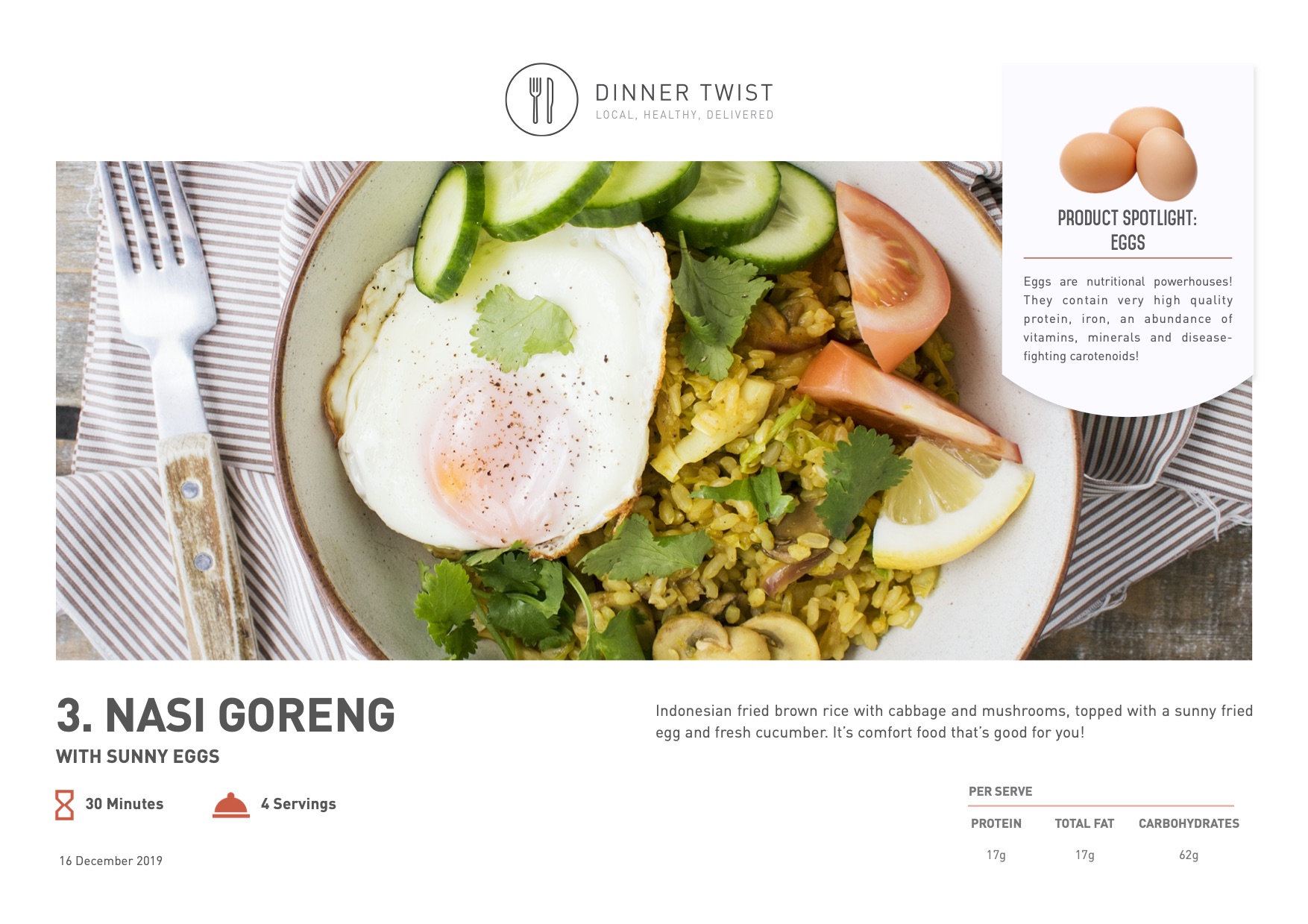The image showcases a webpage from a food advertisement website. At the top, the website's name, "Dinner Twist," is displayed in plain font, accompanied by an illustrated fork and knife inside a circle to the left. 

Below the header, there is an enticing image of a food meal labeled as "Nasi Goreng with Sunny Eggs." The plate features a delicious serving of rice accompanied by sunny-side-up eggs and fresh cucumber slices. A fork with a stylishly shaved wooden handle is placed to the left of the plate, resting on a brown-striped napkin. 

In the top right corner of the image, there is a highlighted section labeled "Product Spotlight" featuring three brown eggs. The text informs viewers that eggs are nutritional powerhouses, providing high-quality protein, iron, and a wealth of vitamins, minerals, and disease-fighting carotenoids. 

Below this description, another subtitle reads "Indonesian fried brown rice with cabbage and mushrooms topped with a sunny fried egg and fresh cucumber." The caption emphasizes that this dish is comfort food that’s also nutritious, boasting a nutritional breakdown of 12 grams of protein, 12 grams of total fat, and 62 grams of carbohydrates.